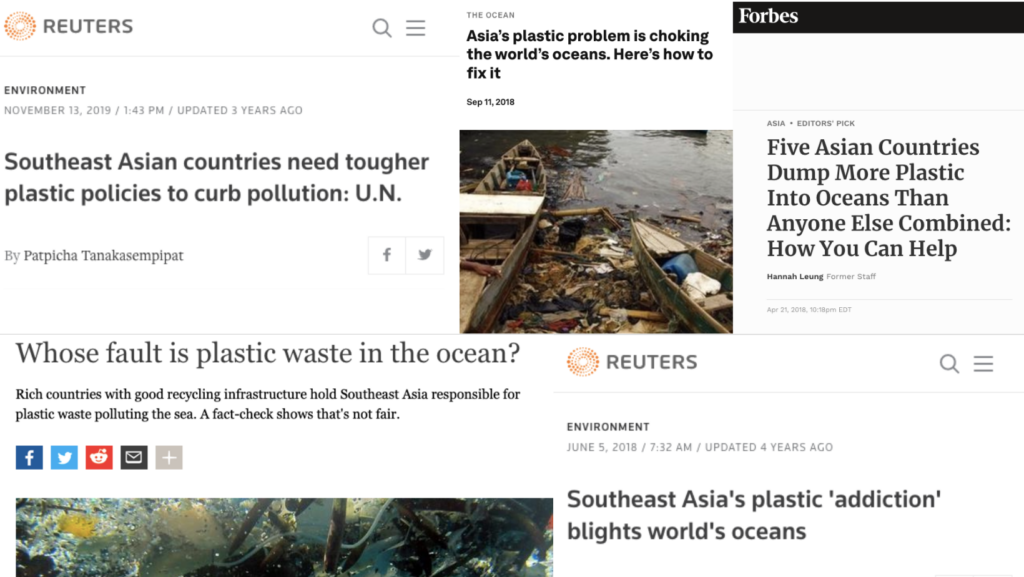The image is a meticulously compiled screenshot taken from a news site, displayed in landscape mode. This collage features multiple news articles side by side, each highlighting the severe issue of plastic pollution in Southeast Asia. 

In the upper left corner, an article from Reuters, under the Environment section, dated November 13, 2019, at 1:43 p.m. and updated three years prior, emphasizes the need for tougher plastic policies in Southeast Asian countries to combat pollution, according to the UN.

Moving to the top center, a piece focused on "The Ocean" discusses Asia's plastic problem and its detrimental impact on the world's oceans. Dated September 11, 2018, the article includes a distressing image of heavily polluted water between two small boats.

In the upper right corner, a Forbes article, tagged under Asia Editors' Pick, points out that five Asian countries contribute more plastic to the oceans than all other countries combined, and offers ways for individuals to help address this issue.

The bottom left corner features a discussion on the accountability of plastic waste in the ocean, questioning the blame placed on Southeast Asia by richer countries with better recycling infrastructures. This section concludes with social media icons (Facebook, Twitter, Reddit, and email) and has a plus button. There's also an accompanying image depicting murky pollution.

In the bottom right corner, another Reuters article from the Environment section, dated June 5, 2018, and updated four years earlier, critiques Southeast Asia's plastic addiction and its dire consequences for the world's oceans. This comprehensive montage was last modified in 2022, offering a stark visual and informational representation of the ongoing plastic pollution crisis.